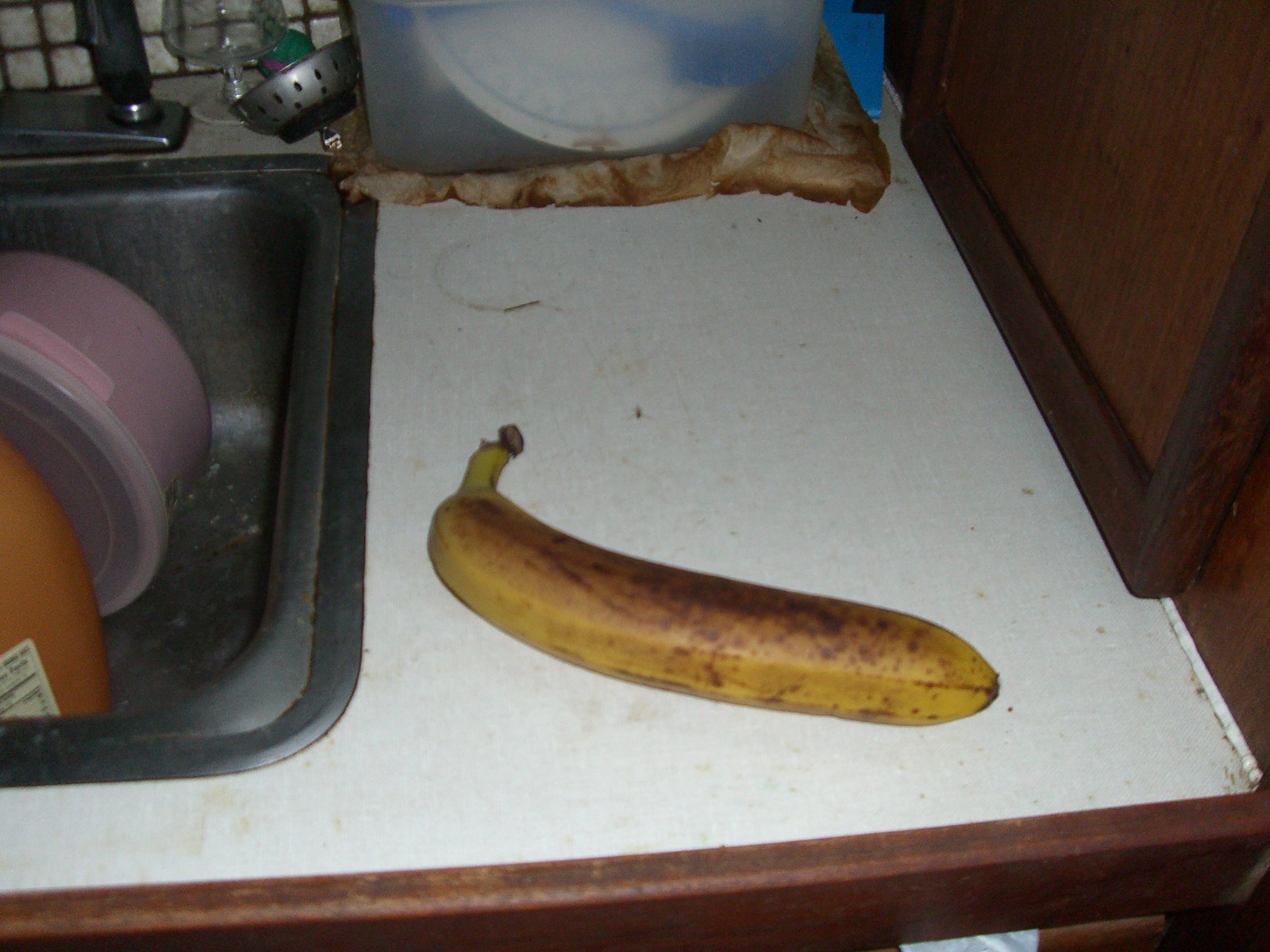The image captures a disheveled kitchen scene with a focus on an aging banana. The banana, speckled heavily with brown spots, is placed at a slight angle on a filthy white counter. This counter, bordered by a wooden edge, highlights its grime through stark contrast. Adjacent to the counter on the right are wooden cabinets adding to the cluttered environment. In the background, a stained brown paper towel lies beneath a plastic tub, which holds a white plate with a blue rim. 

To the left rests a silver sink in dire condition, filled with a pink, round Tupperware container and a partially visible plastic juice jug with a white label. The sink itself is marred with dirt both in and around it. Partially visible in the top left corner is a disconnected silver faucet with a black sprayer, surrounded by dirt and grime. Beside it, a brandy glass and a silver sink stopper add to the disarray. The backsplash, composed of small white tiles, reveals heavily soiled grout, completing the chaotic kitchen setting.